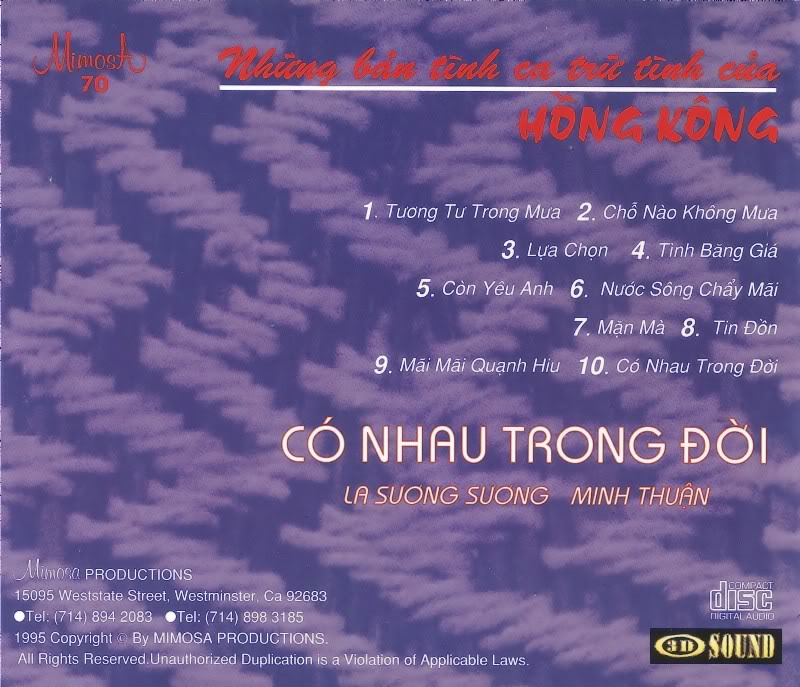The image is a detailed screenshot of a CD album cover, featuring a vibrant color scheme with a blue and purple fabric-like background. The top of the cover displays text in red, written in an unidentifiable foreign language, with the word "Hong Kong" prominently featured in red beneath it. Below this, there is a list of phrases numbered from 1 to 10, each marked with white text, likely indicating the track names. Further down, additional text appears in the same foreign language, presented in a larger white font followed by a smaller phrase. 

In the lower left-hand corner, the cover includes the logo for Mimosa Productions, along with the address, phone number, and a 1995 copyright notice, emphasizing that unauthorized duplication is a violation of applicable laws. The bottom right-hand corner features two mini logos indicating the album’s format: "3D sound" and "compact disc digital audio." The overall design incorporates a mix of light purple, dark purple, red, white, bronze, and gold colors, creating a visually striking advertisement or album cover from 1995.